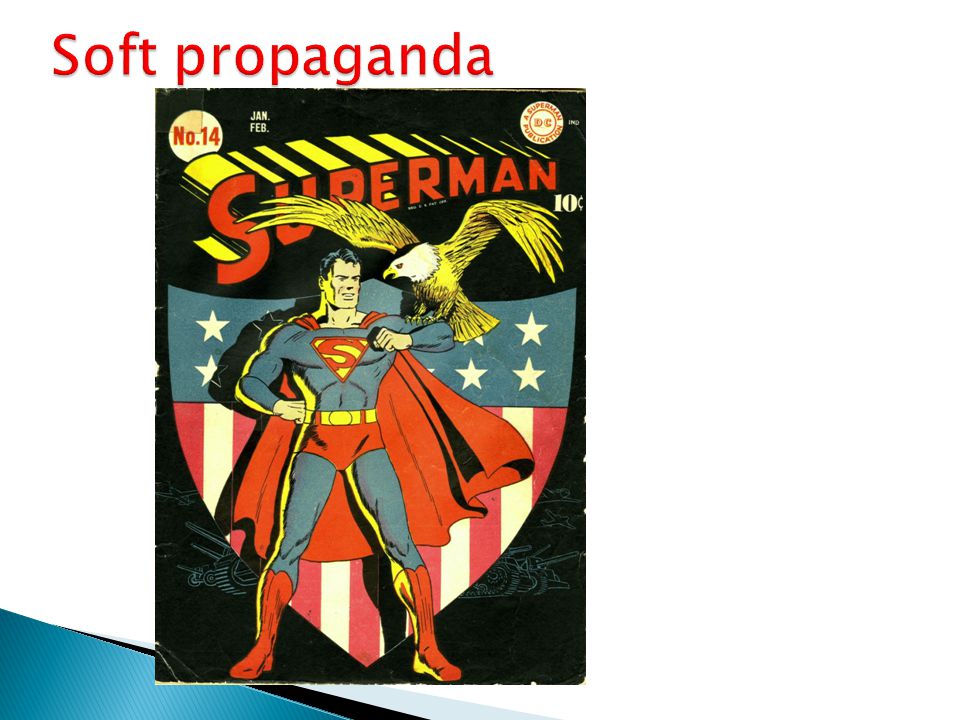The image is the cover of the 14th issue of a Superman comic book. In the upper left corner, the words "soft propaganda" are written in red ink, with the 'S' capitalized. Additionally, there's a yellow circle with "No. 14" written in red, indicating the issue number. Next to it, small white text denotes "Jan. Feb.", marking the publication months. In the upper right corner, a white circle with red letters reads "DC," symbolizing DC Comic Publications, and under it, "10 cents" denotes the comic's original price.

The title "Superman" stands prominently at the top in 3-D red and yellow block letters. Below the title, Superman stands heroically with legs spread, a fist on his waist, and his other arm extended, holding an eagle with a yellow body and beak, and a white head. Superman is clad in his classic blue bodysuit with a red 'S' on his chest, red boots, red "underwear" over his suit, and a yellow belt. A red cape flows behind him, and he stands in front of a large shield bearing the colors and design of the American flag. The overall color scheme prominently features red, blue, yellow, and white, reinforcing the patriotic theme.